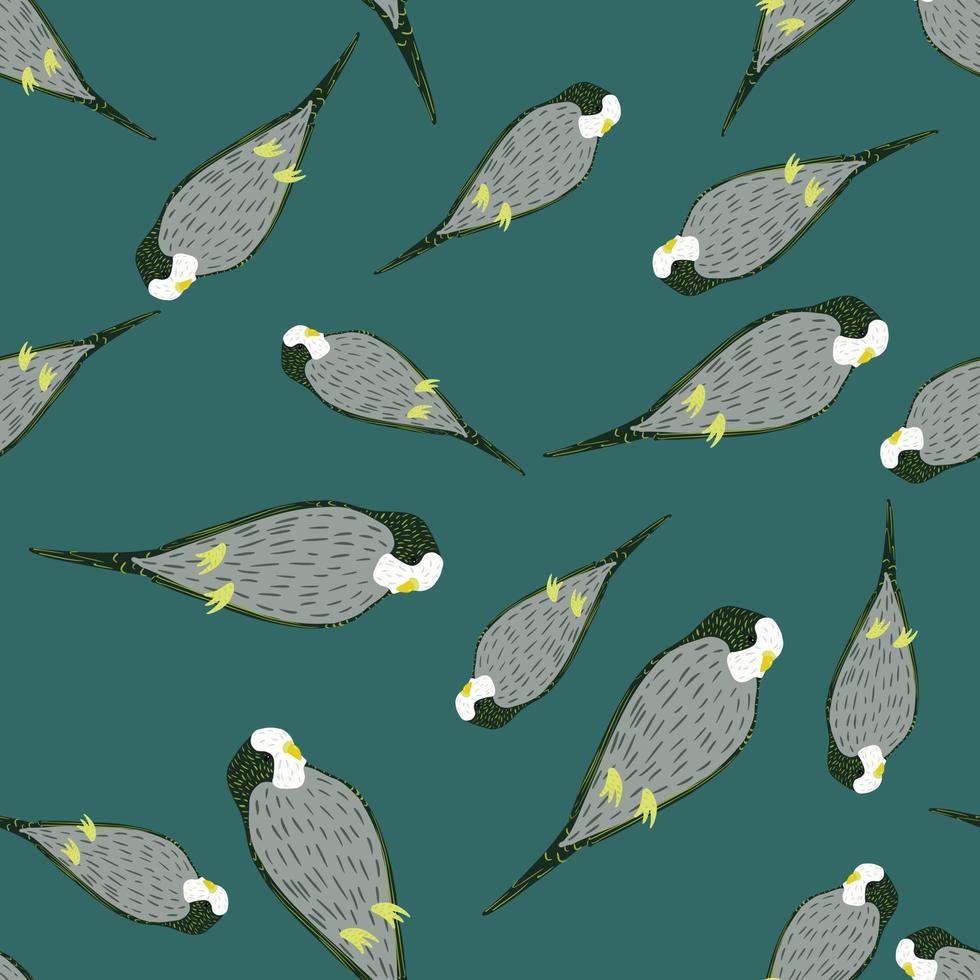This image, reminiscent of a wallpaper design or a painting, features a slightly greenish teal background that sets the stage for a series of small, stylized birds. The birds, varying subtly in size but identical in shape, are scattered across the canvas in different orientations—upright, upside down, and horizontal. Each bird presents a consistent color scheme with a gray body adorned with black lines indicative of feathers, a white face, a yellow beak, and matching yellow feet. Their wings are folded down, giving them an oval or circular appearance accentuated by a pointy tail. The pattern lacks intricate detail but offers a repetitive, decorative motif that's suitable for a fancy wallpaper catalog or as a unique background for a creative project.